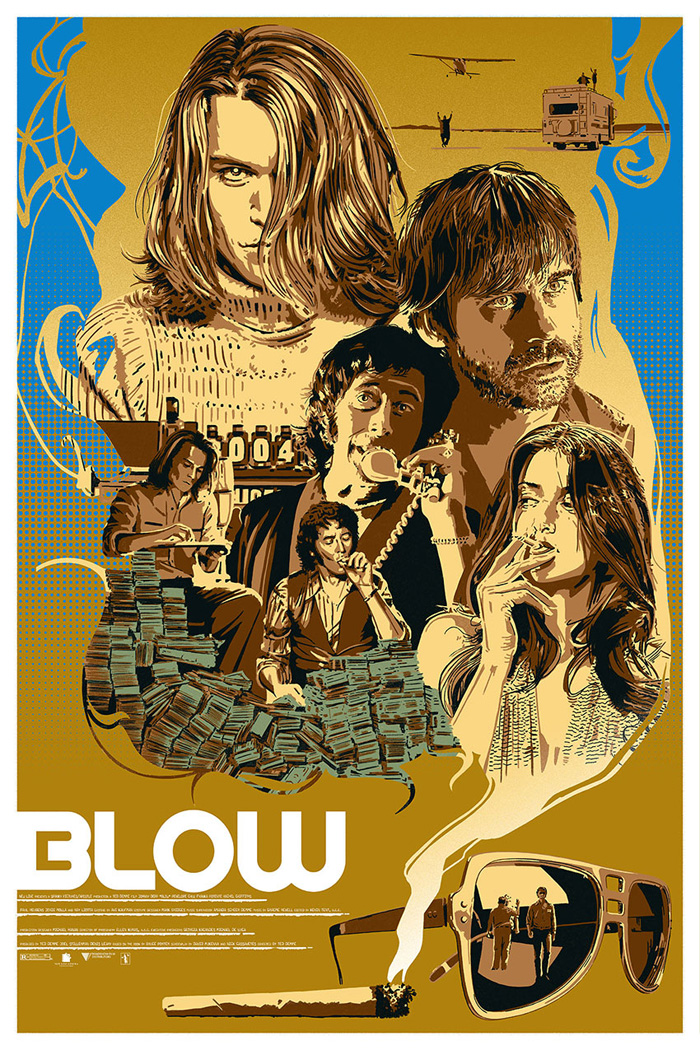The movie poster for "Blow" features a stylized 70s comic book-style illustration. Dominating the bottom left corner, the title "BLOW" appears in bold, white block letters, with smaller, unreadable text beneath it. A lit, smoking cigarette on the left extends its smoke upward, which intricately details various scenes and characters. Within the smoke, there are several figures: a woman smoking, a young man with a shocked expression and stubble, a man in a vest smoking beside a large pile of money, and another man sitting at a desk writing. Further up, a larger man talks on the phone, and a woman with long hair cascading over her left eye stares directly forward, her figure imposing above all. The backdrop of this depiction includes an RV camper in a desert setting on the right and an airplane coming in from the left, with a man waving at it. The lower right corner of the poster showcases mirrored sunglasses reflecting two police officers, adding an intriguing detail to this elaborate digital drawing.